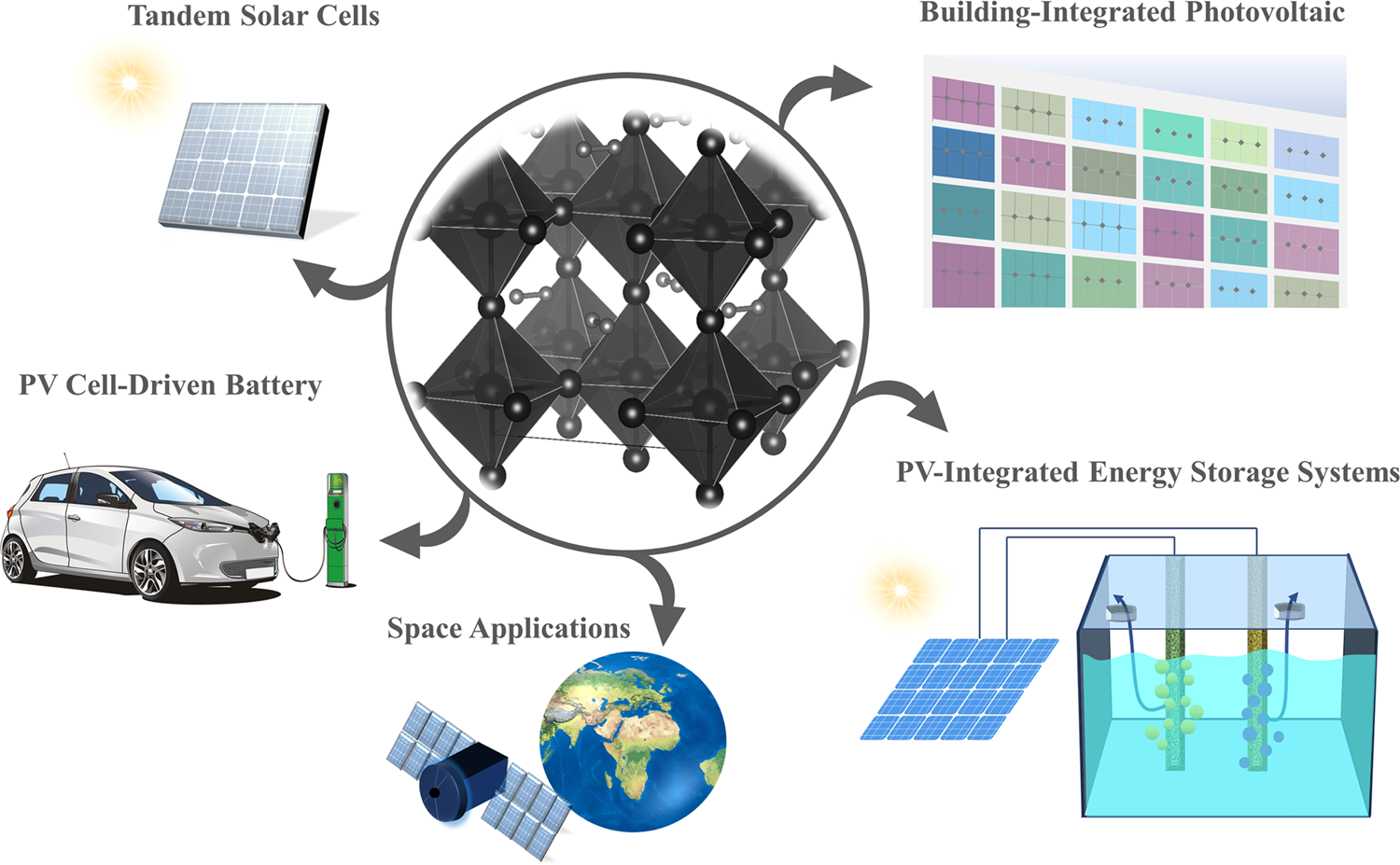This detailed black-and-white graphic centralizes a complex photovoltaic structure composed of interconnected eight-sided geometric forms, resembling dual pyramids joined at their bases. Surrounding this core, five arrows extend outward, each leading to a distinct application of photovoltaic technology. The top right arrow points to "Building Integrated Photovoltaics," featuring images in muted colors. Below it, the "PV Integrated Energy Storage Systems" displays solar panels powering a submerged device. Directly at the bottom, "Space Applications" is illustrated by a satellite orbiting Earth. The bottom left arrow denotes a "PV Cell Driven Battery," showcasing an electric car being charged. At the top left, "Tandem Solar Cells" completes the circle. Each pointed-to image provides either a diagrammatic representation or a realistic example of these varied photovoltaic applications.